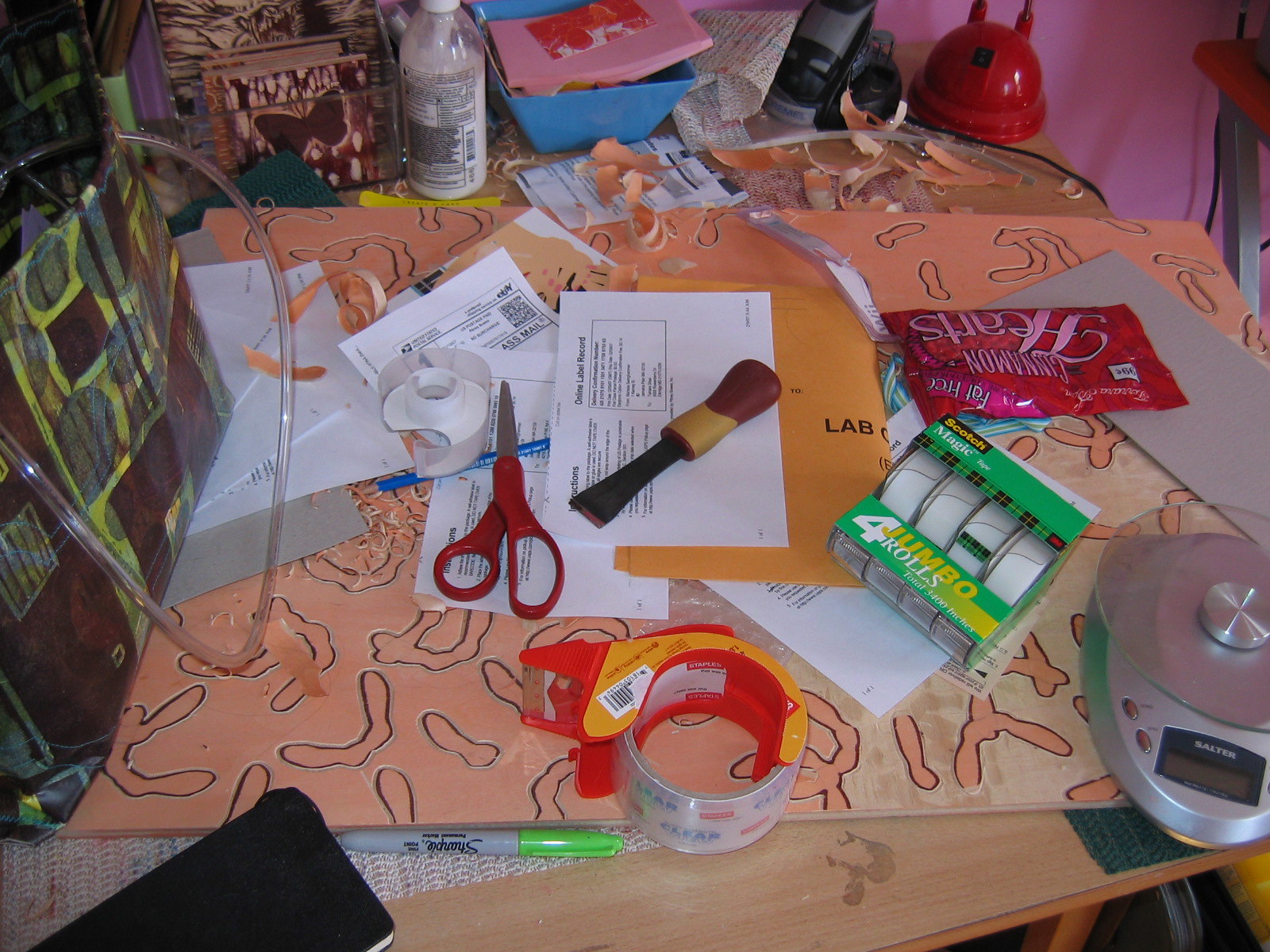The image depicts a cluttered table, the surface of which appears to be faux wood. Dominating the table is a piece of wood intricately etched with various leaf patterns resembling oak and poplar leaves in diverse shapes and sizes. Atop this wooden piece sits a jumbo four-pack roll of Scotch tape. 

In the lower right corner of the table, a food or package scale is positioned, while a Moleskine notebook lies in the lower left corner. Scattered around the table are various items, including a fluorescent green Sharpie and a roll of packing tape situated centrally. 

On the extreme left side, there is a brown vinyl bag adorned with green designs. Additional items include a pair of scissors, a chisel-like tool, an envelope, an eBay mailing label with instructions, and a tube of hand cream.

Towards the back of the table, a lamp and another appliance, possibly a wood shaver, can be seen. A blue plastic square bowl containing random pieces of foam is also visible. At the far back left of the table, a collection of handmade stamps is placed, rounding out the assortment of objects on this busy table.